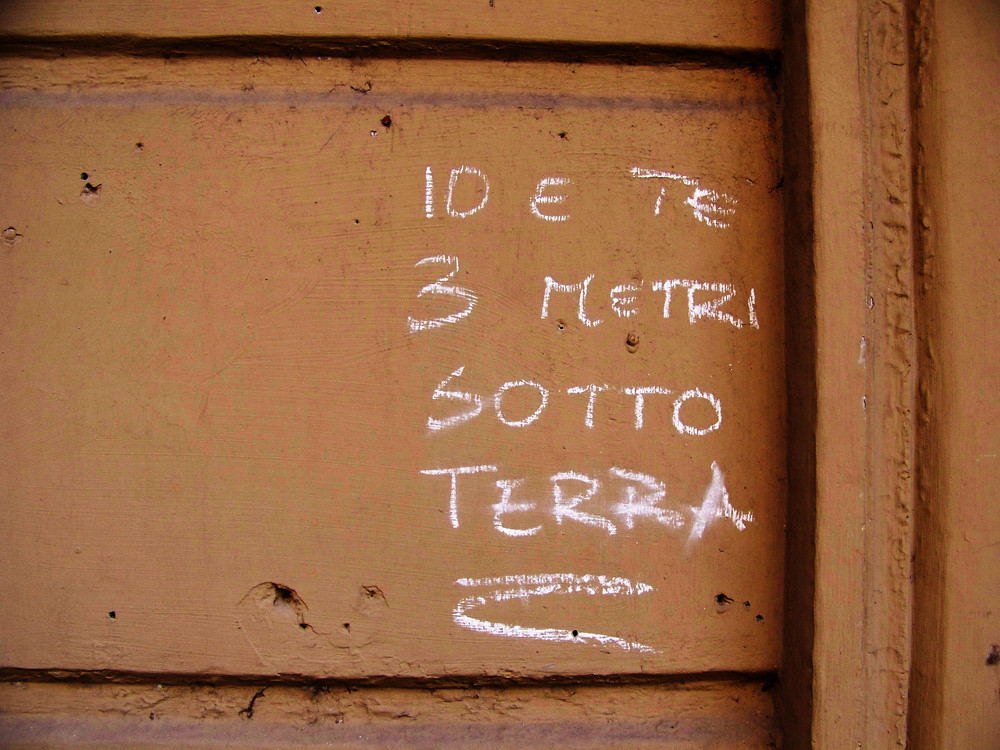The image reveals an up-close perspective of a brownish-orange painted wall that appears to be made of cement. The surface of the wall is characterized by various holes, possibly left behind from previous nails, and features two horizontal lines at the top and bottom, suggesting a construction of stacked rectangular cement blocks. On the central portion of this wall, there is a series of words written in white chalk. The inscription is arranged in four lines: "I-D-E-T-E", followed by "3-M-E-T-R-I", then "S-O-T-T-O", and finally "T-E-R-R-A". Below the last line, "T-E-R-R-A", is a white chalk squiggle. The wall is bordered on the right by identical vertical boards painted in the same brownish-orange color, which frame the overall structure and reinforce the appearance of a solid, foundational wall. Additionally, a subtle purple line traverses the wall's surface, adding a contrasting detail to the otherwise monochromatic palette.